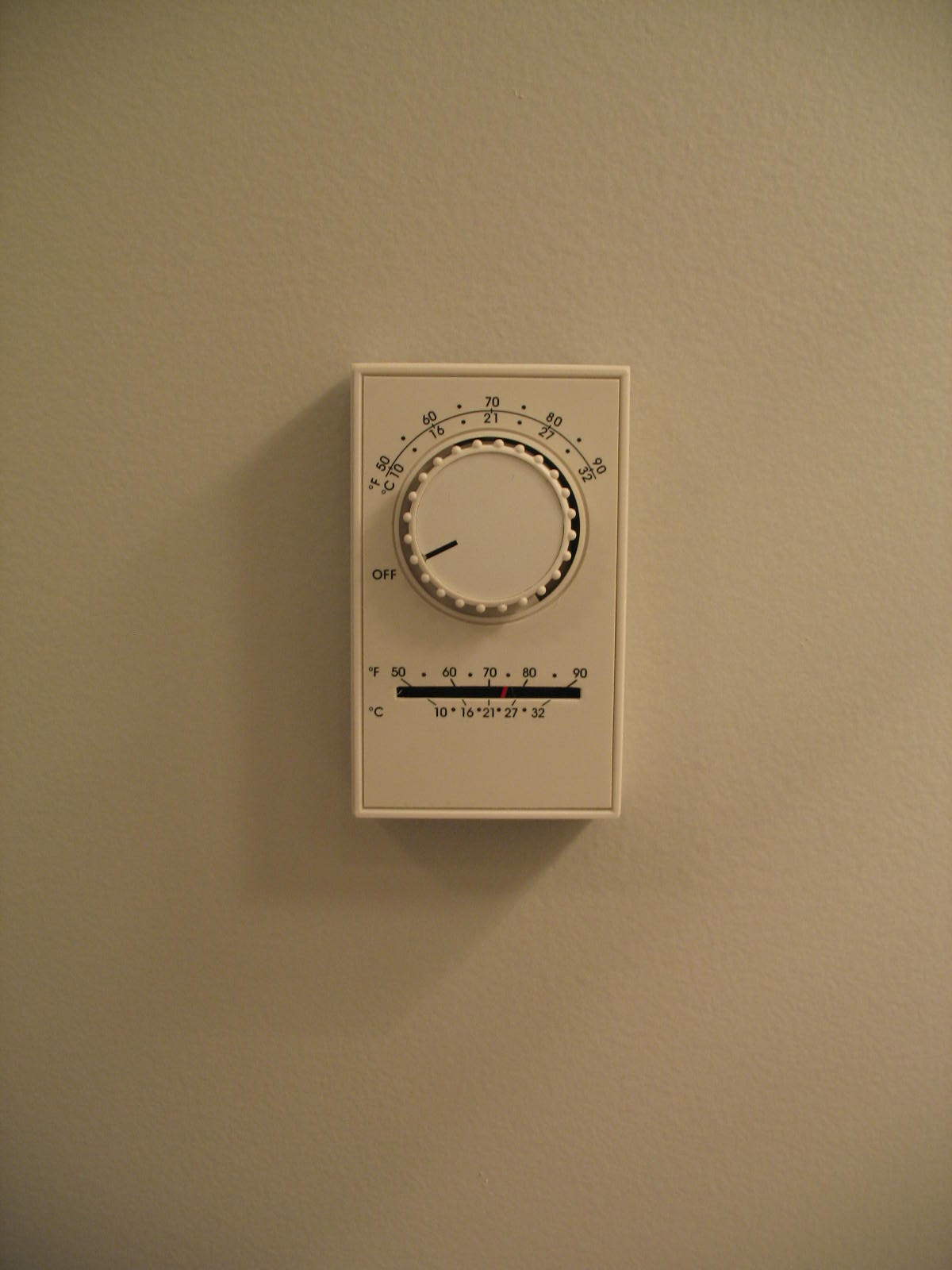This vertical photograph depicts a wall thermostat mounted on a tan-colored wall, blending seamlessly with the background. The rectangular thermostat is captured in a straight-on view, showcasing its minimalist design devoid of any visible manufacturer branding on the front panel. Dominating the upper portion of the thermostat is a large, ribbed dial designed for easy gripping. This dial features two arcing scales—Fahrenheit above and Centigrade below—ranging from the "off" position at approximately the 8 o'clock mark to 90 degrees Fahrenheit at around the 2 o'clock mark. Below the dial is a smaller, rectangular opening with an additional scale, also measuring in both Fahrenheit (on top) and Centigrade (below), presumably for fine-tuning the temperature settings.